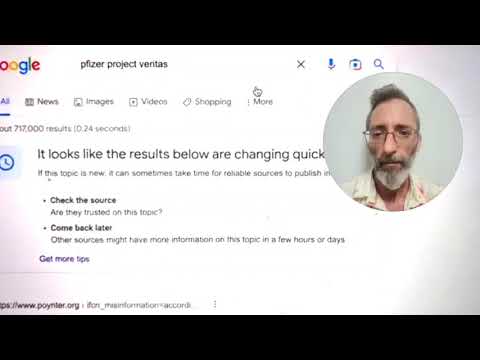The image is a nearly square screenshot of a Google search page, bordered by elongated horizontal black bars on the top and bottom, reminiscent of a widescreen format. The search engine's distinctive logo appears at the top, though the "G" is cut off, showing only "oogle" in its characteristic red, yellow, blue, green, and red letters. The search query displayed in the search bar reads "Pfizer Project Veritas." Central to the image, in prominent text, is a notification stating "It looks like the results below are changing quickly," with smaller bullet points advising users to "Check the source" and to "Come back later." In the upper right corner, encased in a circular frame, is a photograph of an older white male. He has short, slightly curled gray hair, glasses, a gray and white beard, and a mustache that transitions into a goatee. He wears a collared shirt that's partially unbuttoned, revealing a bit of his chest, and stands against a plain white background.